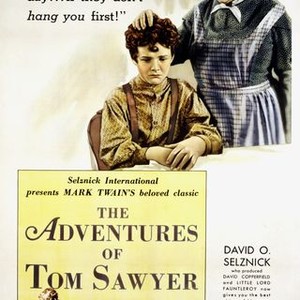The image is a partial view of a vintage-looking book cover or poster for "The Adventures of Tom Sawyer," presented by Selznick International. The illustration prominently features a boy, possibly Tom Sawyer, dressed in an old-fashioned yellow dress shirt and overalls with overall straps. He is sitting in a chair, facing forward with his hands clasped together, and appears to be pouting. Behind him, a woman whose head is not visible—suggested to be his mother, as she is wearing an apron with black and light blue stripes—places her hand gently on his head. The backdrop has a distressed, yellowish-white square that states in black print: "Selznick International presents Mark Twain's beloved classic, The Adventures of Tom Sawyer." Adjacent to this, in black text, it reads: "David O. Selznick, who produced David Copperfield and Little Lord Fauntleroy," with more text that is not fully readable. Above the boy’s head, partially visible black text shouts, "Hang You First!" giving an added dramatic flair to the scene. The image has a nostalgic, old-time feel, reminiscent of an advertisement or a book cover from another era.